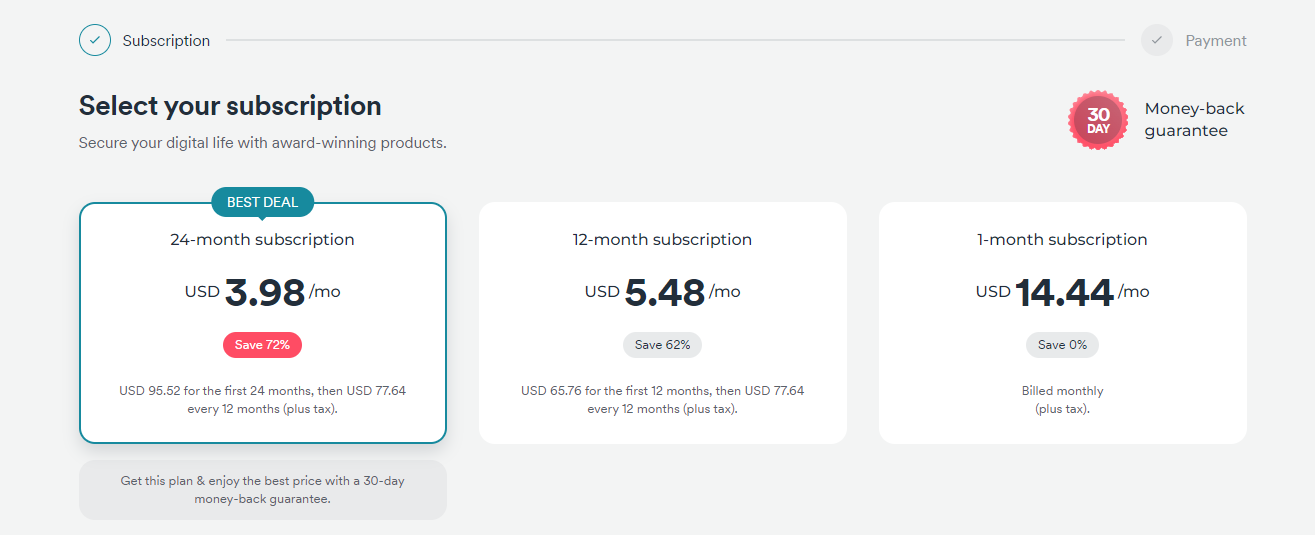In the image, there is a horizontally elongated gray rectangle. On the upper left corner, a green-outlined circle with a green check mark inside it is found, accompanied by the word "Subscriptions." A gray dividing line separates this section from the right side, where another circle, gray in color with a darker gray check mark, is placed next to the word "Payments" written in gray.

Below this header, toward the left, there is a large black font title that reads "Select Your Subscription." Underneath it, in smaller gray font, is the phrase "Secure your digital life with an award-winning product."

Three white rectangular product options are displayed in a row beneath this text, each longer on the horizontal axis. The first product is highlighted as "Best Deal," with this label enclosed in a green and white outline. The details inside this first rectangle state: "24-month subscription, USD $3.98/mo, Save 72%" in an oval red background. It further specifies, "USD $95.52 for the first 24 months, then USD $77.64 every 12 months, plus taxes."

Adjacent to the first option, the second product offers a "12-month subscription" at "USD $5.48/mo, Save 62%." It goes on to mention, "USD $66.75 for the first 12 months, then USD $77.64 for every 12 months, plus tax."